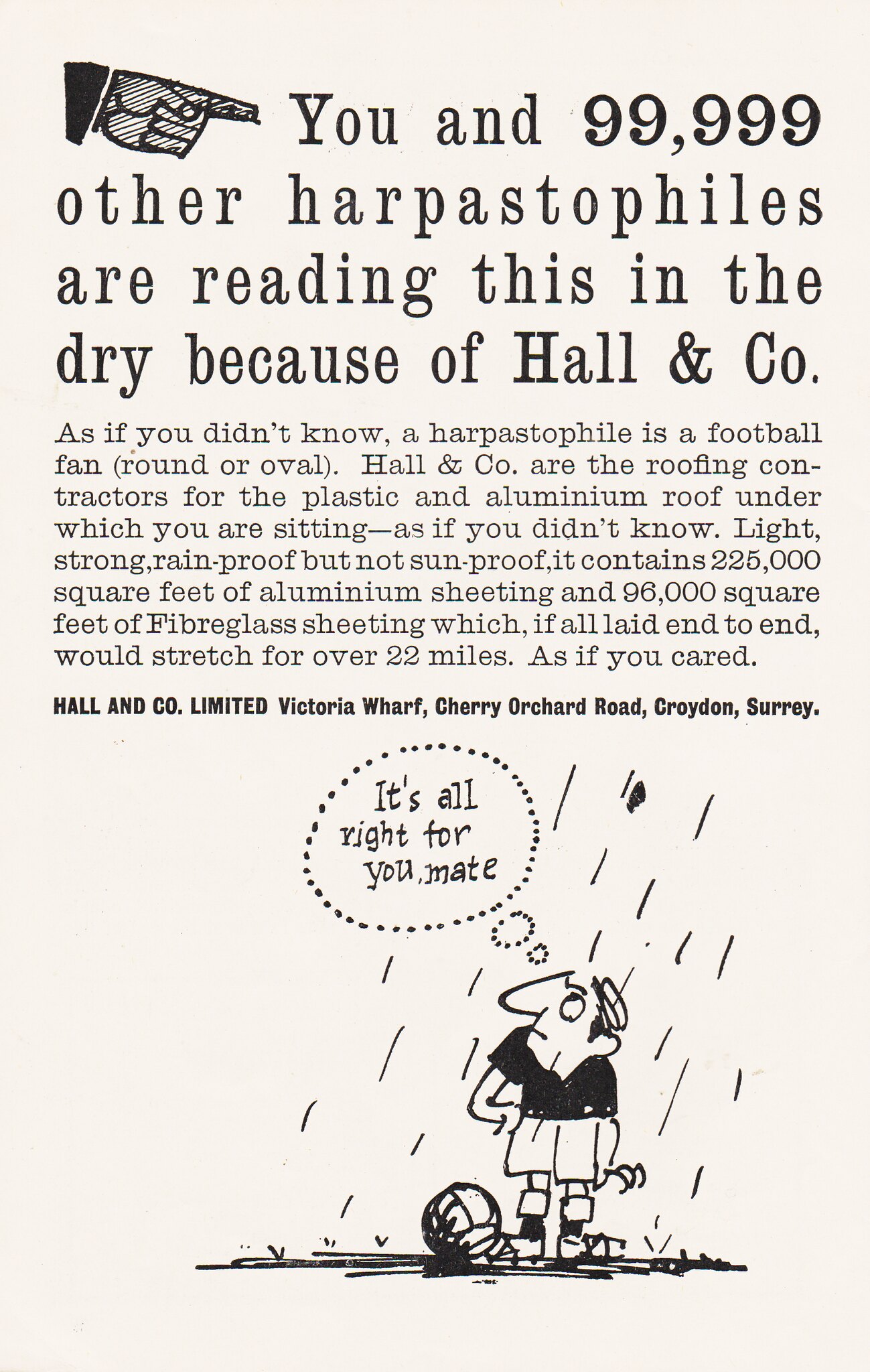The image, presented on an off-white or beige background, features a cartoon at the bottom and accompanying text in black font. At the top left corner, a sketch of a hand with the index finger pointing introduces the text that reads, "You and 99,999 other harpestophiles are reading this in the dry because of Hall & Co." The term "harpestophile" is defined as a football fan, whether fan of round or oval games. Hall & Co. are credited as the roofing contractors for the plastic and aluminum roof under which the reader is sitting. The roof is described as being light, strong, rainproof, but not necessarily sunproof, boasting 225,000 square feet of aluminum sheeting and 96,000 square feet of fiberglass sheeting. If all the materials were laid end-to-end, they would stretch over 22 miles. The detailed description concludes with the company's address: Hall & Co. Ltd., Victoria Wharf, Cherry Orchard Road, Croydon, Surrey. Below this text, the cartoon depicts a soccer player standing in the rain, looking upwards, with a speech bubble that reads, "It's all right for you, mate." The soccer ball is at his feet, rain pours down, and the ground is visible.